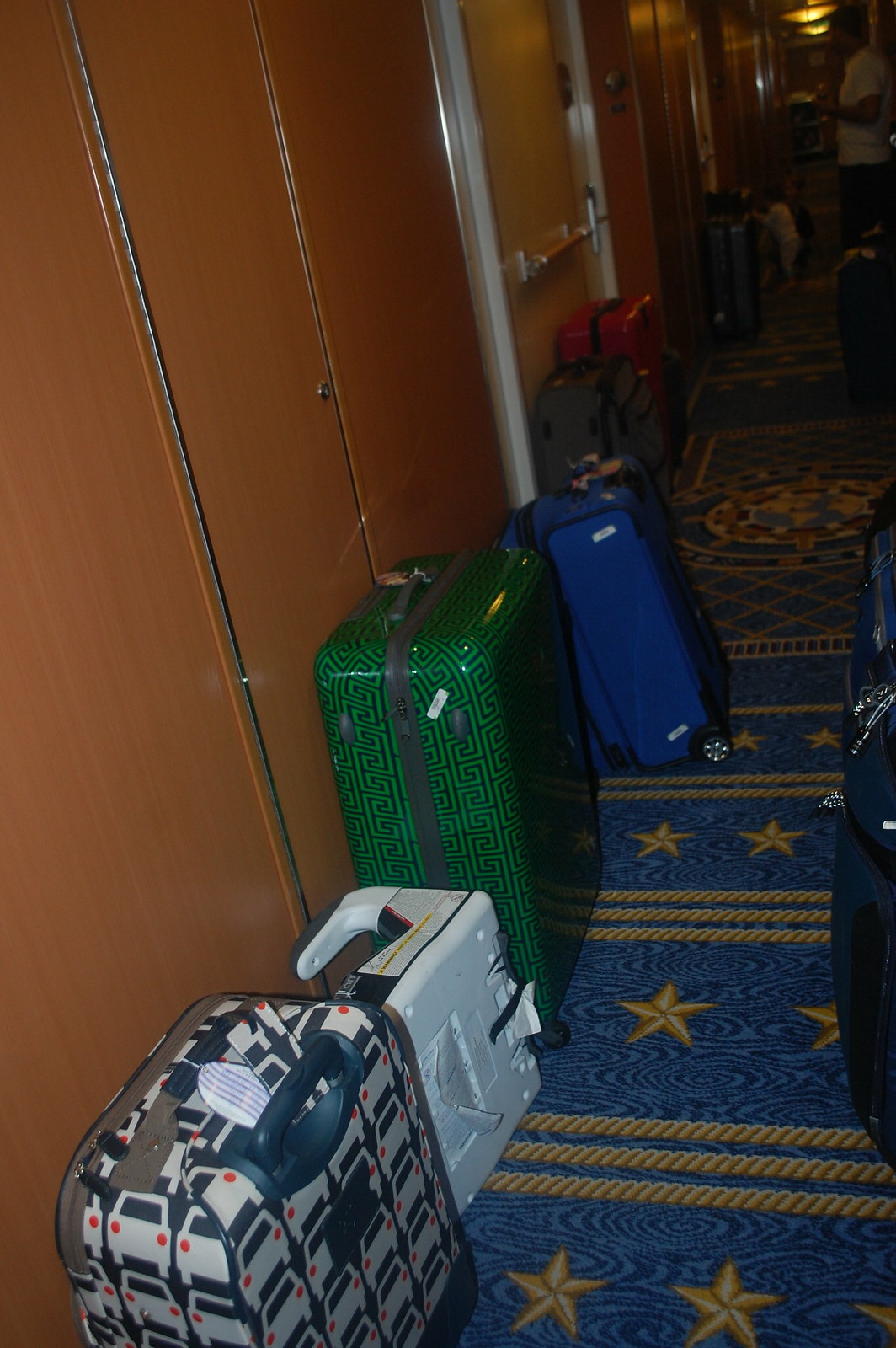This portrait-oriented photograph captures an assortment of suitcases and luggage in a long hallway, reminiscent of an 1980s or 1990s design, potentially located within a cruise ship or hotel setting. The hallway features a distinctive blue rug with a repeating pattern of gold stars and three gold stripes, enhancing a nautical theme. Leaning against a brown wooden wall are four suitcases: one black-and-white with red headlights in a car pattern, a white one, a bright green piece with Givenchy logos, and a blue nylon bag. Extending further into another room, visible through the hallway, there are additional gray and burgundy suitcases on a blue, diamond-shaped rug. The scene includes a man standing to the right, with people, possibly a woman and child, further down the hallway. In the background, exit and cabinetry doors add to the structural detail, hinting at a functional yet nondescript environment.